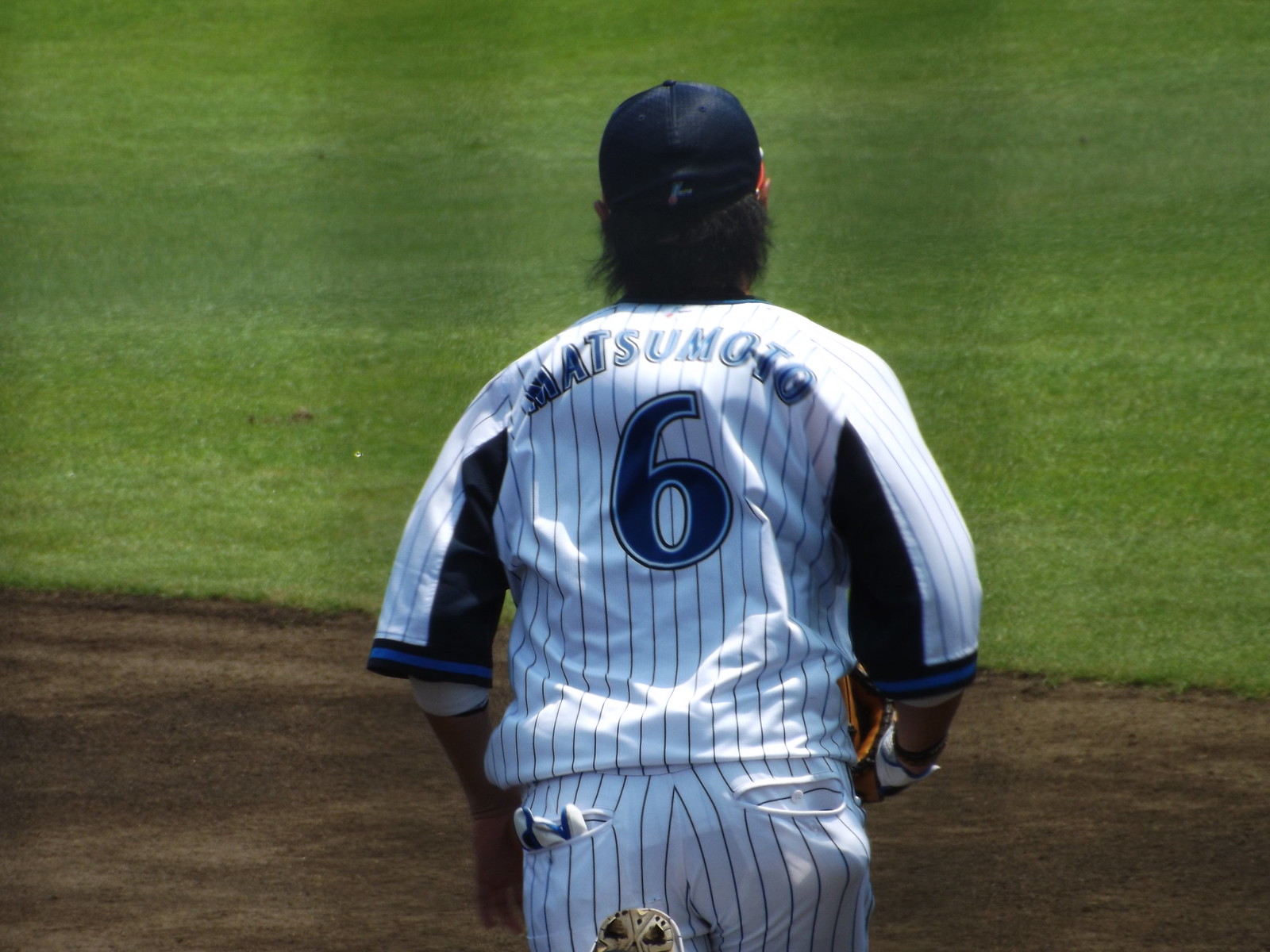The image captures a rear view of a baseball player poised to run onto the field. His body is shown from just below the waist up to the top of his head. The player is on the edge of a dirt infield, with the majority of the background being lush, short-cut green grass. His outfit consists of a white uniform with blue pinstripes, featuring the number six prominently on his back, above which is his last name, possibly "Matsumoto," although the exact spelling is unclear. His sleeves end at the elbows and are bordered with black-blue-black trim, and he is equipped with two white elbow pads. He wears a black hat with some light blue writing that is not fully legible. His jet-black hair, reaching his shoulders, extends from under the cap. In his right hand, he carries a baseball glove, partially visible in front of him, while another glove's tips peek out from his back left pocket. The scene is set on a well-maintained field with a clear demarcation between the grass and the dirt infield.